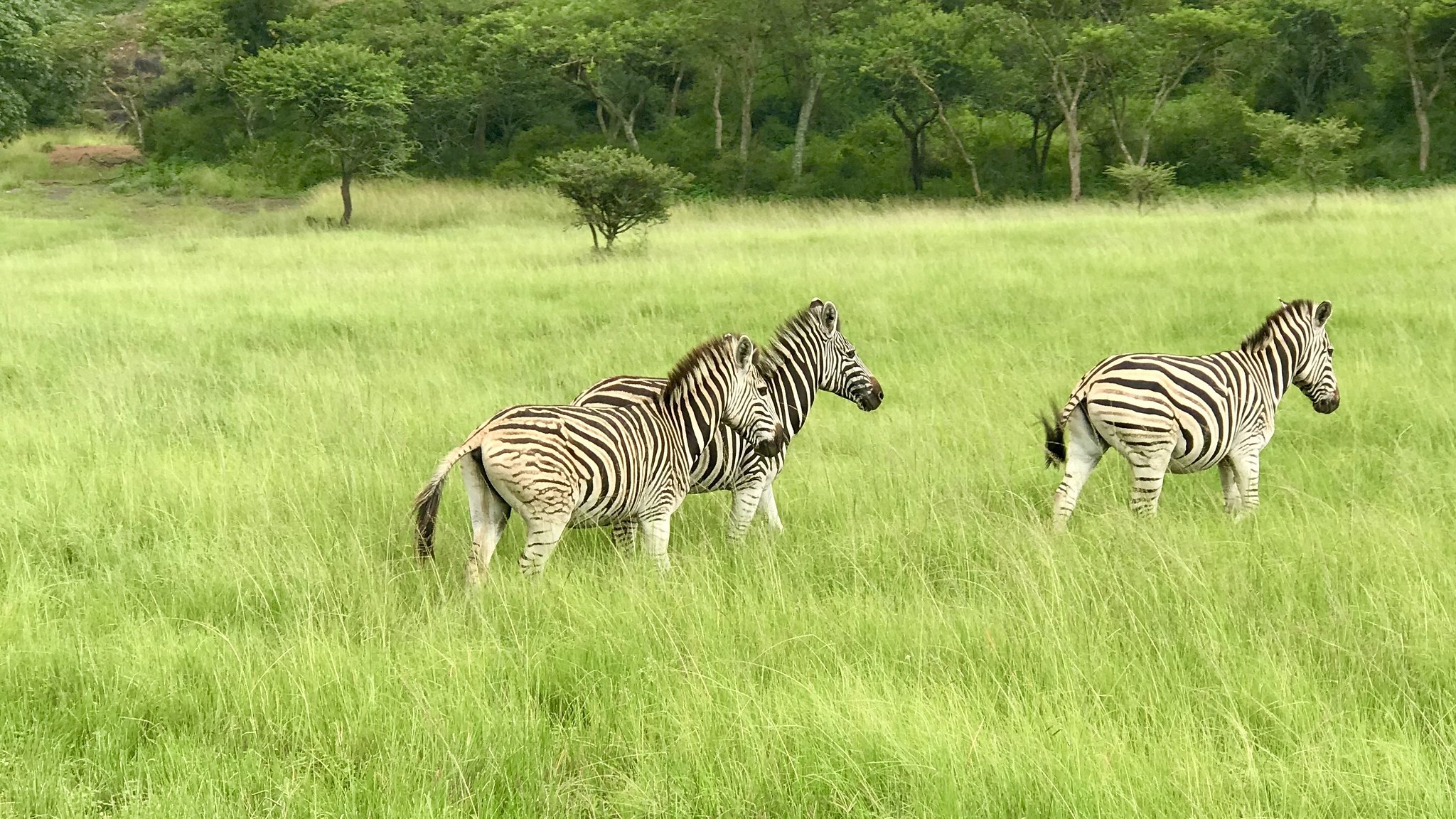This is a color photograph taken outdoors, showcasing three zebras walking through a densely packed, tall grassy field. The grass has a uniform appearance, predominantly yellow-green, reaching up to the zebras' bellies, and rippling gently, possibly due to the wind. The zebras' striking coats feature black and white stripes with black manes and tails adorned with a long black fringe. Two zebras stand closely together while the third is slightly to the right, all moving from left to right. They are facing right, and one zebra is captured flicking its tail, possibly to ward off flies. In the background, taller and denser green trees with brown trunks form a contrasting backdrop to the lighter, softer hues of the grassy field, enhancing the natural beauty of the scene.